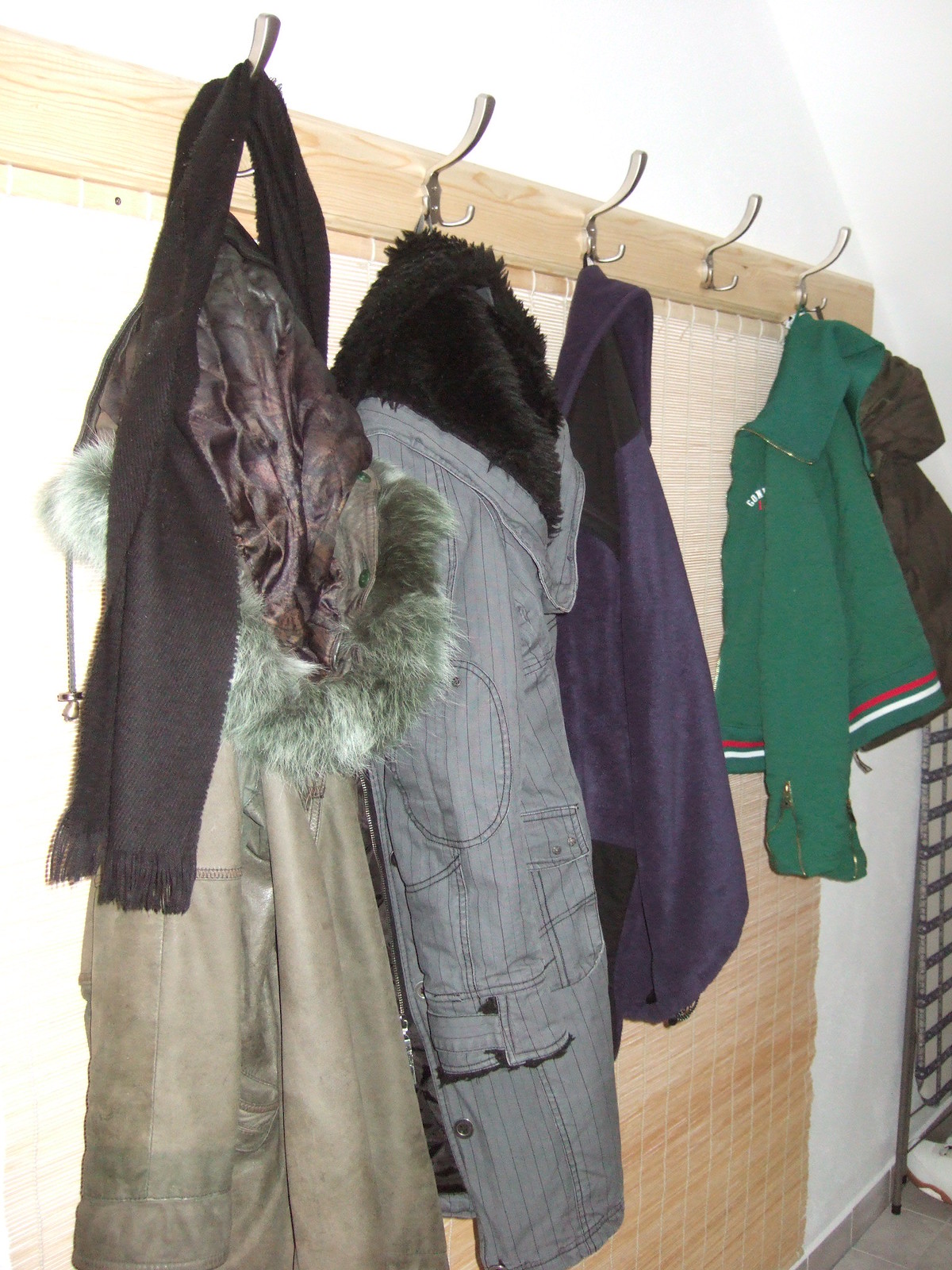The image depicts a wall-mounted coat rack viewed from a slight left-hand angle, giving a diminishing perspective of its contents. The rack, which is secured to the wall by a light brown wooden board, is adorned with five silver hooks, though the fourth hook remains unused. 

Hanging prominently on these hooks are four various coats and a black scarf. Starting from the left, the closest and largest garment due to the perspective is a light green coat with a hood, draped over with a black scarf. Next to it, a gray coat featuring a black furry hood occupies the subsequent hook. Adjacent to this, a plush, purple fleece coat is on the third hook. The fourth hook is empty, and the fifth hook supports a green baseball-style jacket that features red and white stripes at its bottom hem, beside which hangs a brown coat. Additionally, an indistinct black object is partially visible to the far right of the image.

These items, hanging from distinct metal hooks affixed to the wooden strip, suggest a domestic setting, reinforced by the cozy and varied materials of the coats.